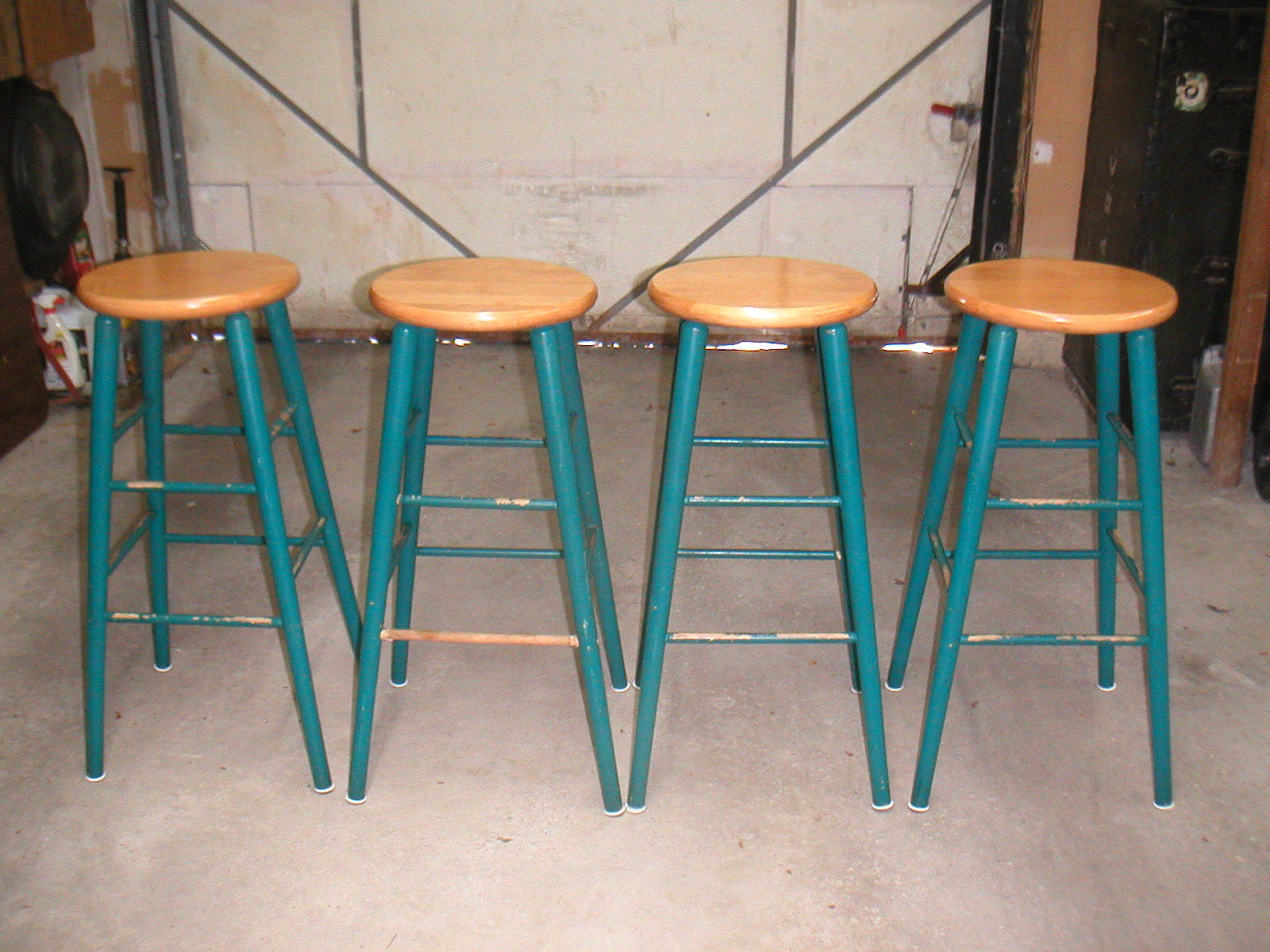This photograph features four bar stools arranged in a line, situated within what appears to be a garage or workshop area. The stools boast highly varnished pine seats, circular in shape, perched atop legs painted in dark turquoise. The paint on the legs is chipped in multiple places, revealing patches of the underlying wood. The background showcases a white wall adorned with gray, V-shaped, and vertical lines, resembling the mechanism of a garage door. To the top left, a bag and a shovel are partially visible. The floor is composed of gray cement, speckled with darker gray and reddish spots. This image appears to be a listing photograph, possibly for sale on an online marketplace, capturing the stools in a somewhat distressed yet functional condition.